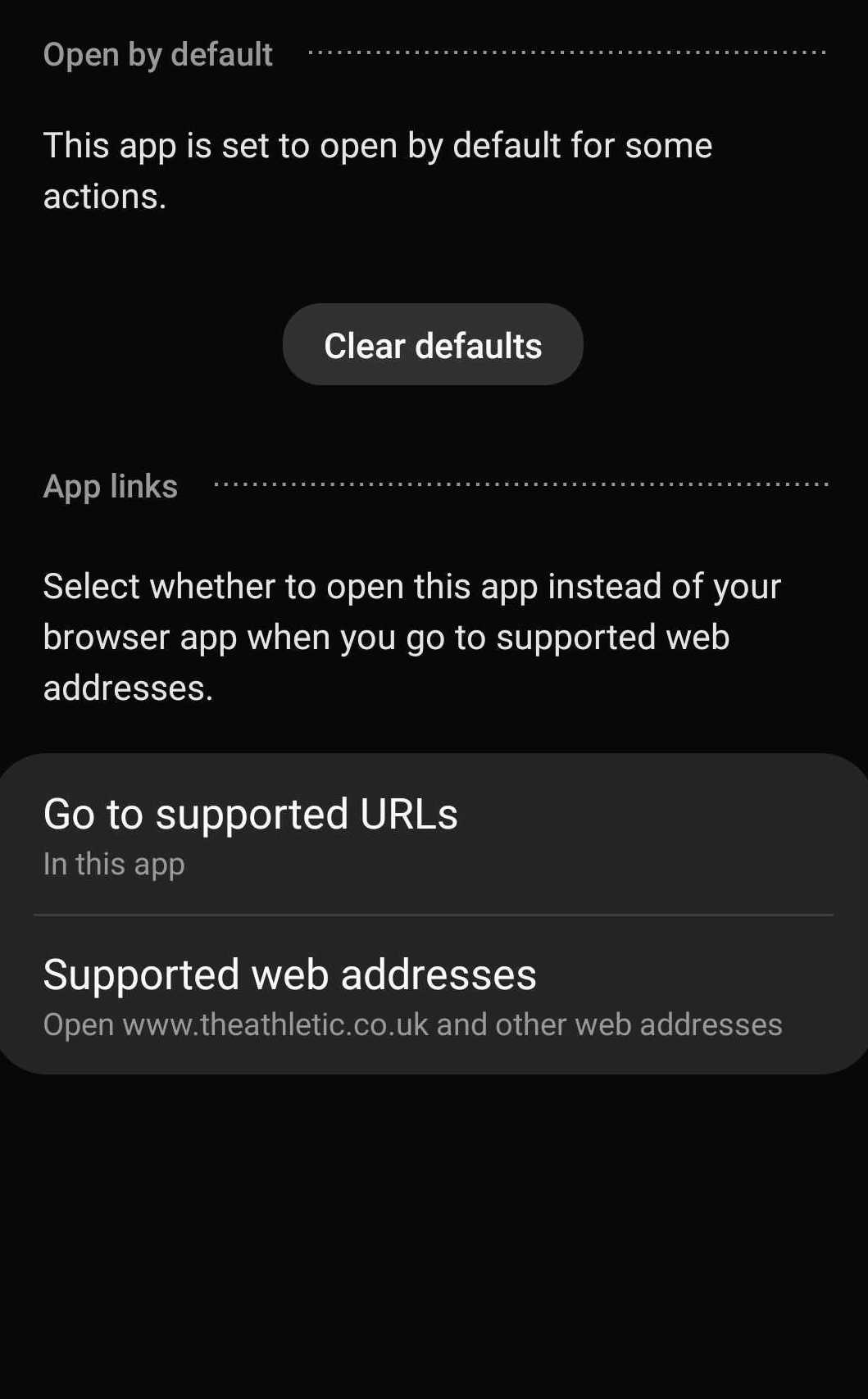The image showcases a dark-themed settings page on an Android phone, specifically within an app's configuration menu. The top section displays options for setting the app as the default for certain actions, with a "Clear Defaults" button readily available. Scrolling down, there's an "App Links" section where users can choose whether to open supported web addresses in this app rather than their default browser. Users can select the "Go to supported URLs" option to dictate that these links open "in this app." Supported web addresses include domains like theathletic.co.uk among others. The page is organized with perforated lines between sections, enhancing readability and navigation through the settings. This detailed view allows users to specify how specific web content is handled by their Android device, demonstrating customizability for a streamlined user experience.